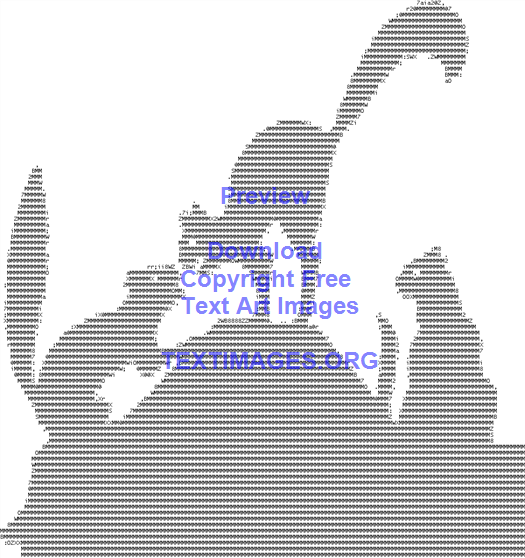The image appears to be a digitally created graphic on a white background, constructed in a dot matrix or pixel art style. Central to the composition are three black, squirrel-like animals, arranged distinctly on a truncated pyramid or mound structure. The leftmost squirrel stands on the base, facing the middle squirrel, which is positioned atop the mound with its tail arched high and back arched downward toward the left squirrel. The rightmost animal, which seems less squirrel-like and more potentially cat-like, sits observing the interaction between the other two, with its tail raised high. Superimposed over this entire scene in blue text are the words "preview," "preview," "download," "copyright free," "text art images," and at the bottom, "textimages.org".